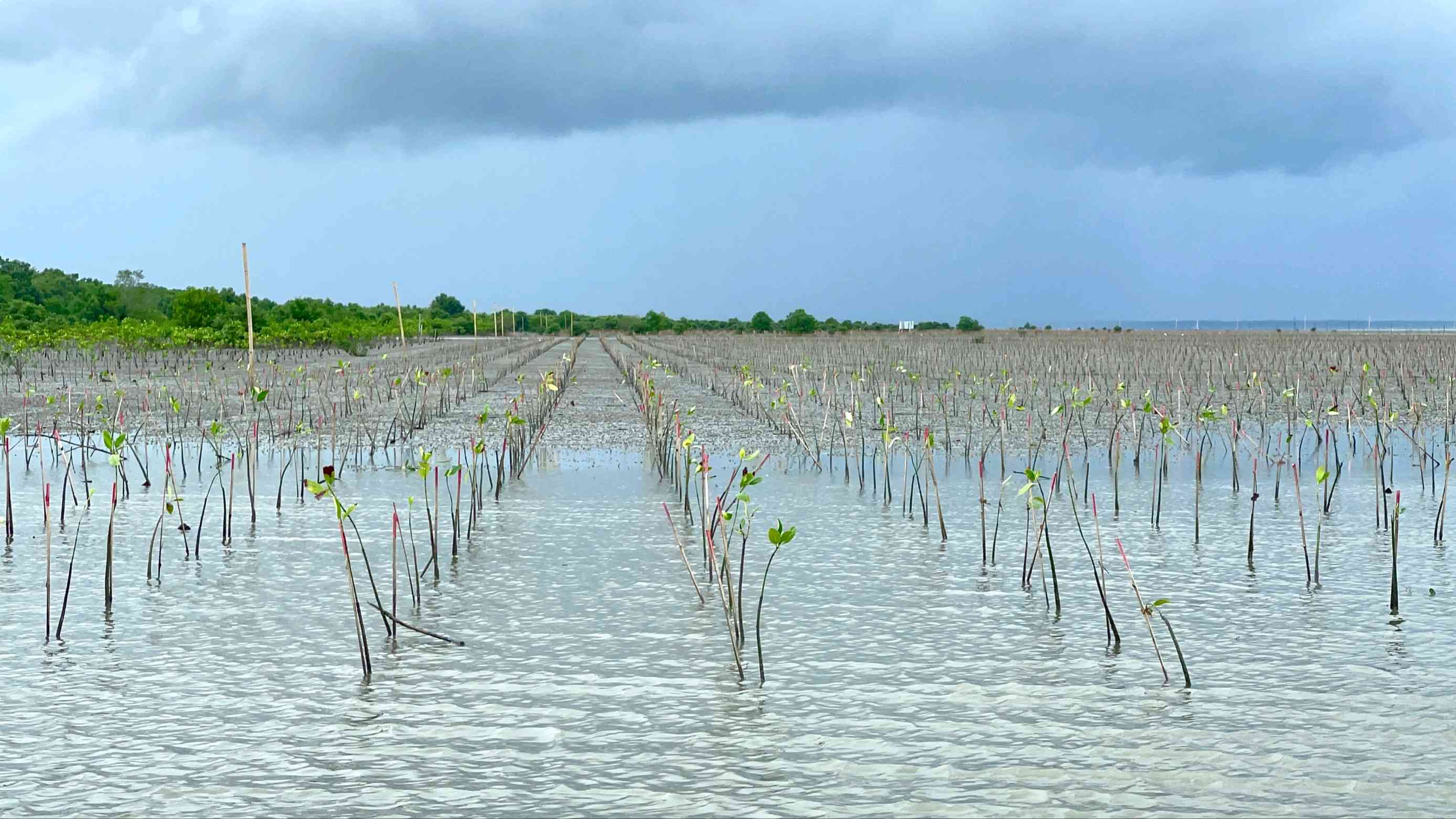This landscape photograph captures a vast, flooded agricultural field, likely rice paddies, stretching across the entire bottom half of the image. The meticulous rows of tall, thin-stemmed plants with green leaves sprouting at the tops create a striking pattern, each standing in shallow water that reflects the overcast sky above. The sky itself dominates the top half of the image, painted in shades of light blue and dark gray, indicating imminent rainfall from the looming, ominous clouds. A strip of lush, green trees extends across the horizon, gradually giving way to the extensive waterlogged field below. The left side of the image features dense shrubbery, adding a varied texture to the scene, while the right side opens up more visibly to the planted rows. The overall atmosphere is serene yet foreboding, capturing the raw essence of a countryside landscape on the brink of rainfall.